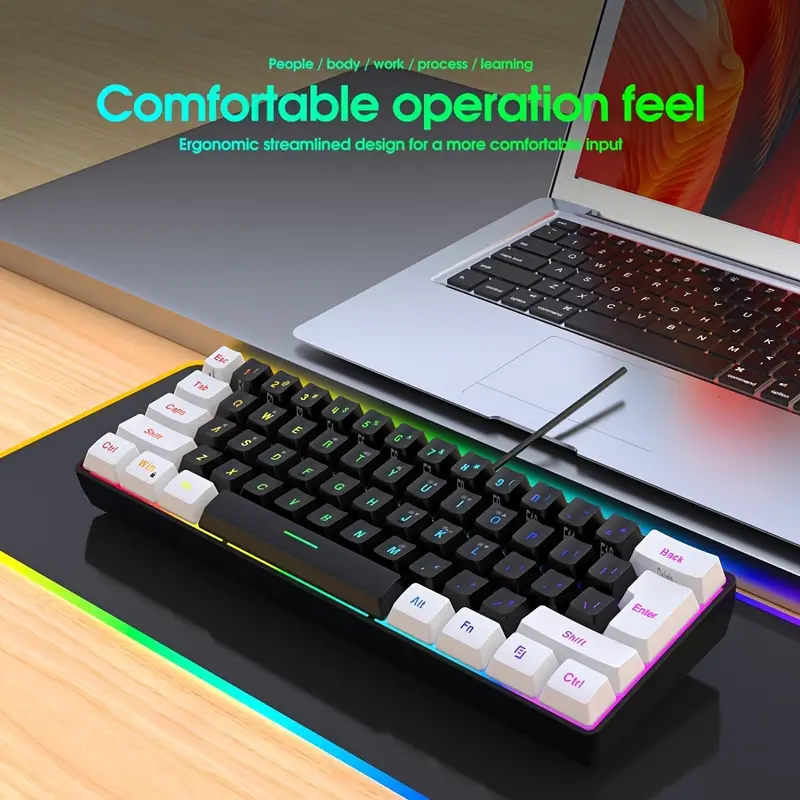The image showcases a tech setup on a brown wooden desk with darker brown lines and grooves. In the top right corner lies a silver laptop with black keys and white text, displaying a vibrant background of orange, white, red, and black. The laptop rests on a silver pad. Below, there is a compact 60% keyboard with a black and white color scheme on the keys, featuring various colored keycaps in red, yellow, green, blue, purple, and orange. The keyboard sits on a black pad encircled by RGB lighting that transitions through yellow, blue, and purple hues. Above the keyboard, an advertisement reads: "people / body / work / process / learning," followed by "comfortable operation feel, ergonomic streamlined design for a more comfortable input," in a gradient from blue on the left to green on the right. The overall setup emphasizes ergonomic design and vibrant RGB aesthetics, highlighting both the laptop and the uniquely illuminated keyboard.